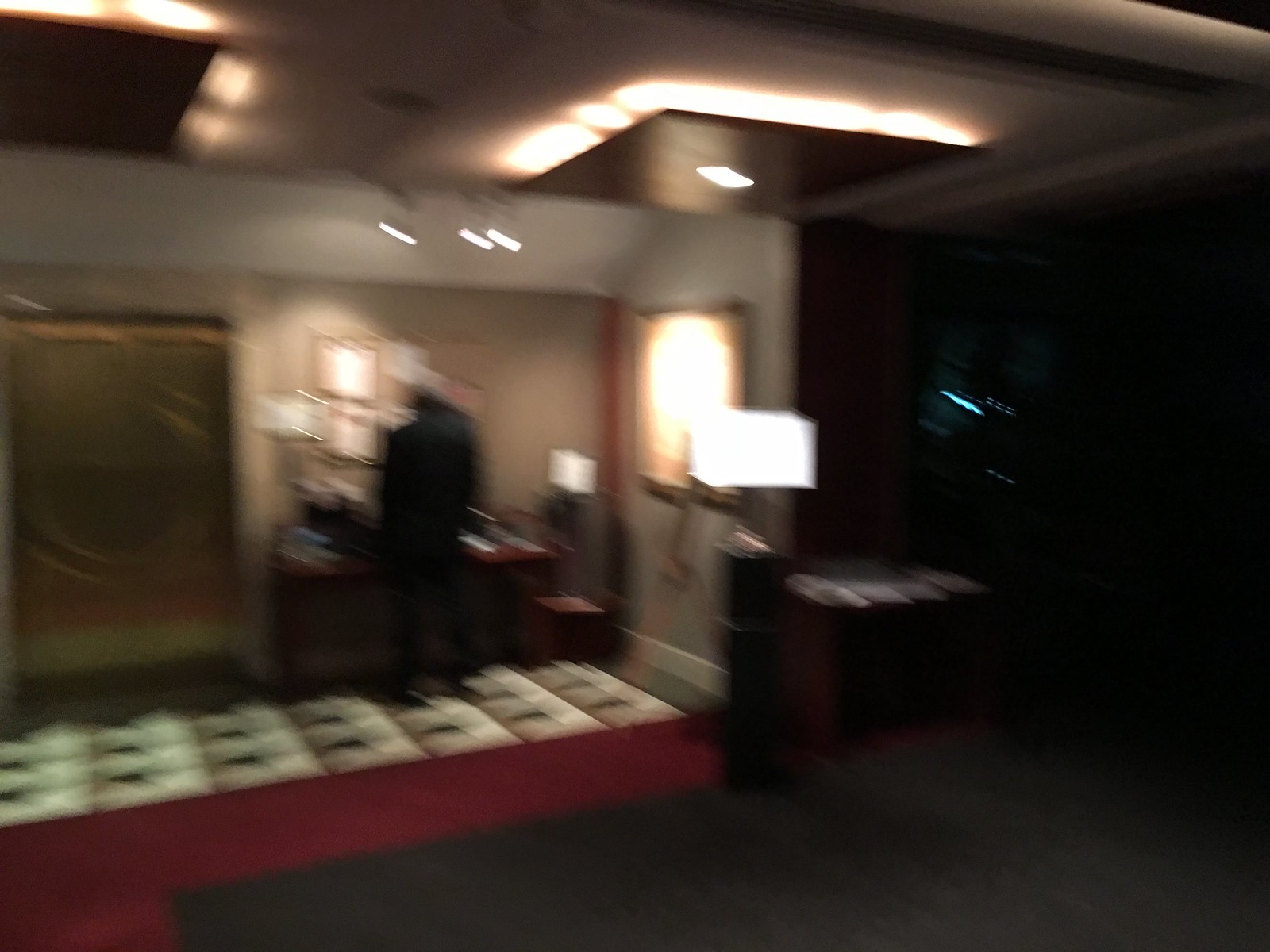The extremely blurry photograph captures an interior room with largely indistinguishable details due to the poor image quality. The room has predominantly gray walls that are intermittently punctuated by various lighted spots or dashes. The ceiling is outfitted with what appears to be a light fixture. In the foreground, there is an object with a red-and-white grid pattern, though its identity remains unclear. The floor features a mix of textures and colors: a red section with a grayish rug and a dark section, possibly black, on the right. In the background, there is a doorway and a tan wall, but these details are not clearly discernible. A person dressed in black stands facing a wall, possibly near a desk which is adorned with picture frames above it. Next to this setup, there might be a table containing white papers and an additional lamp with a white shade. Although many elements in the image, such as a desk and other pieces of furniture, are hinted at, the overall lack of clarity makes specific identification challenging.